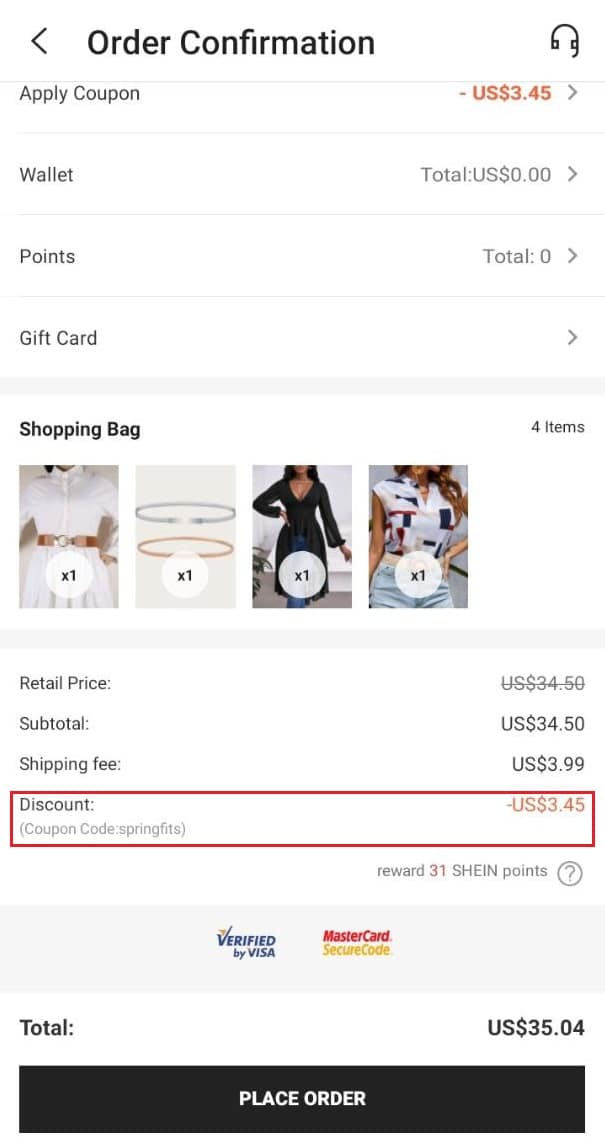A vertical screenshot, likely taken from a mobile device, displays an order confirmation page with a white background. 

At the top of the screen, an arrow pointing left is positioned next to "Order Confirmation." Below this, the phrase "Apply Coupon" is followed by a deduction: "- U.S. $3.45." The "Wallet Total" is shown as "U.S. $0.00," while "Points Total" and "Gift Card" are both marked as zero, with a small right-pointing arrow beside them.

The "Shopping Bag" section indicates there are four items. The images of these items are displayed from left to right, including a white dress, two bracelets (one gold and one silver), a black dress worn by a woman, and a white shirt with a blue and red square pattern, paired with blue jeans.

The retail price of $34.50, crossed out, denotes a discount, bringing the subtotal to $34.50. The shipping fee is listed as "U.S. $3.99," and a discount of "U.S. $3.45" is emphasized in a box with a bold red border. Below this, the reward of "31 shine points" is mentioned.

At the very bottom, a large dark blue or black button labeled "Place Order" invites the user to finalize their purchase.